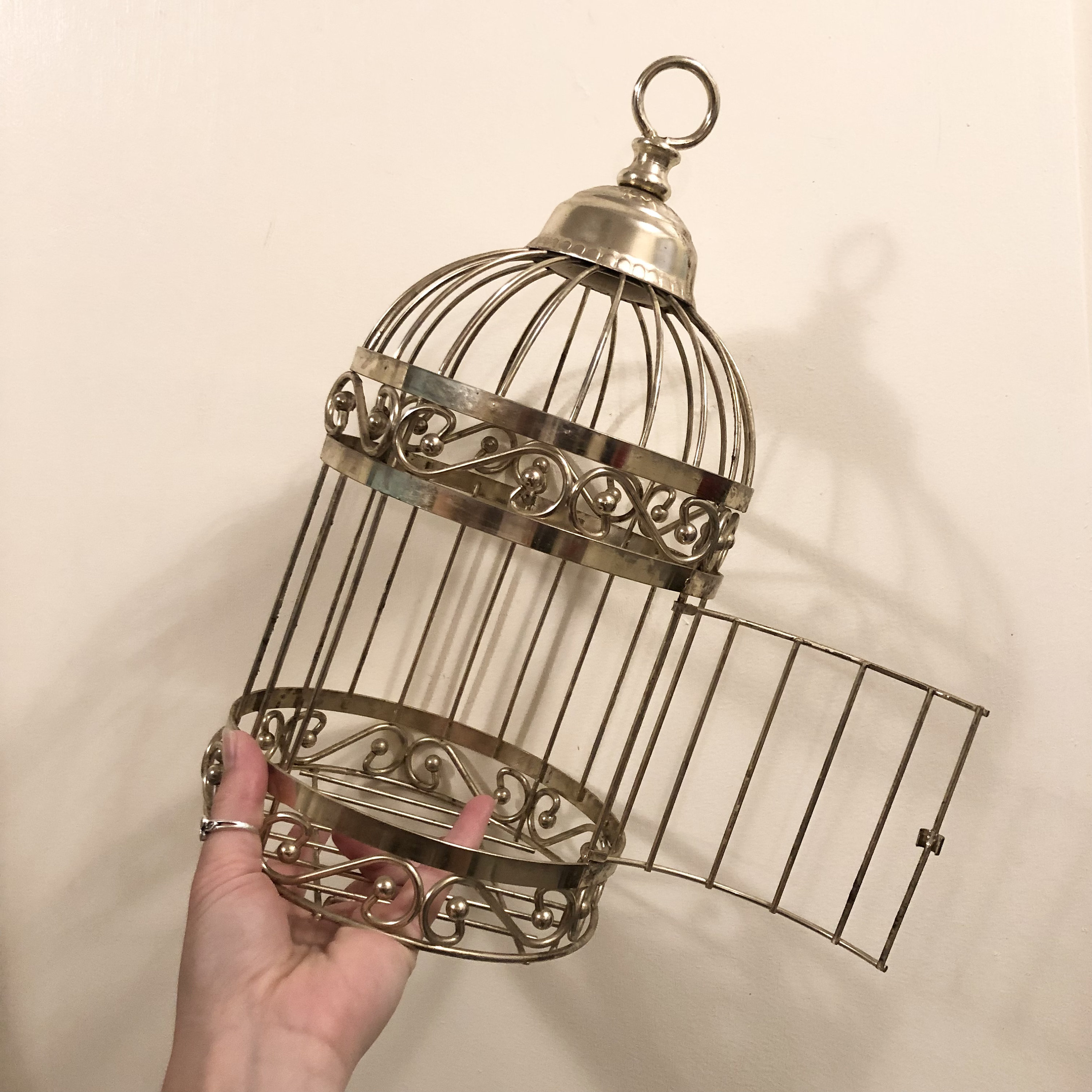In the image, a light-complected woman with a silver ring on her thumb holds a small, decorative metal birdcage against an off-white, cream-colored wall. The birdcage, which has a slightly shiny silver appearance, features intricate decorative bands around its midpoint and base where it starts to curve. It is designed to look like it could hold a candle rather than a real bird. The cage's door is swung open and tilted at about a 35-degree angle, creating a dramatic effect with its shadow cast on the wall behind. The woman's hand, visible from the wrist up, clasps the birdcage from the bottom while her pinky protrudes through the bars. At the top of the birdcage, there is a loop for hanging, suggesting its use as a decorative item. This photograph, capturing the birdcage in such a way, could likely be used for selling the item online.